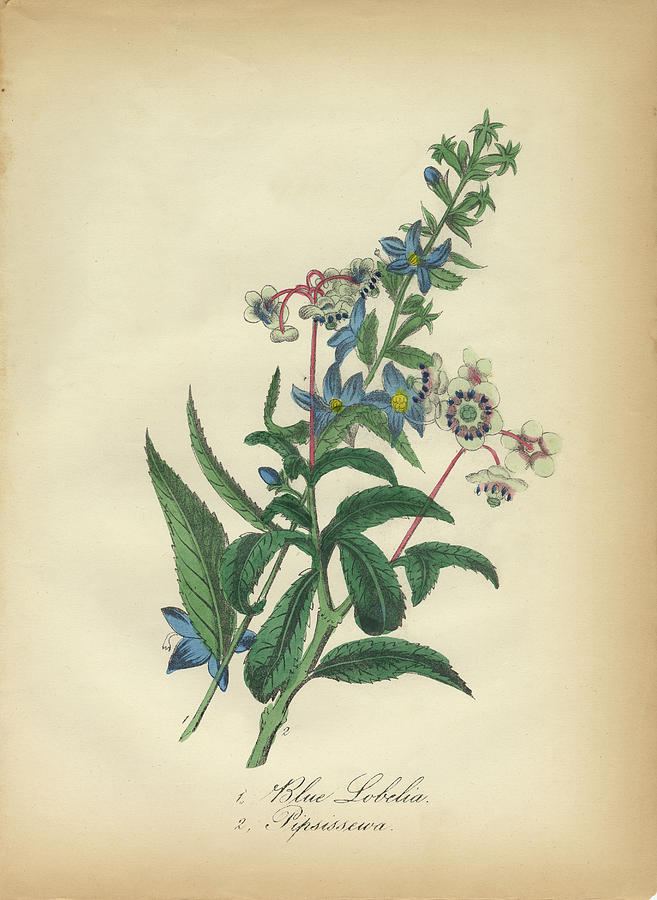This detailed colored drawing appears to be a historical botanical illustration set against a creamy, parchment-like background, evoking the pages of an old book or textbook on horticulture. The vertical-oriented artwork prominently features two distinct wildflower stems, both extending diagonally from the lower left to the upper right corner of the page.

The first plant, identified in the script as "blue lobelia," is characterized by its slender green stem adorned with elongated, jagged-edged leaves. The blossoms, numbering four to five per bloom, are a vivid blue with delicate, narrow petals, and encase a central yellow seed sack. The flowers rest upright on their green stems, presenting a striking contrast to the background.

The second plant, with the partially legible name "pipsissewa," has a similarly long and thin stem, though it transitions to a red hue as it approaches the flowers. The leaves here are also elongated but appear slightly furry or textured. The drooping white flowers crown the red stems, each bloom comprising five petals with pink interiors and a blue central dot, encircling green seed sacks. The presence of these colorful details enhances the intricate design of this botanical piece.

The image is accentuated by handwritten text, likely identifying the species, with "blue lobelia" clearly readable and the second name "pipsissewa" suggested. The details, from the paper-like background to the finely rendered flowers, highlight the artwork's focus on botanical accuracy and aesthetic appeal.